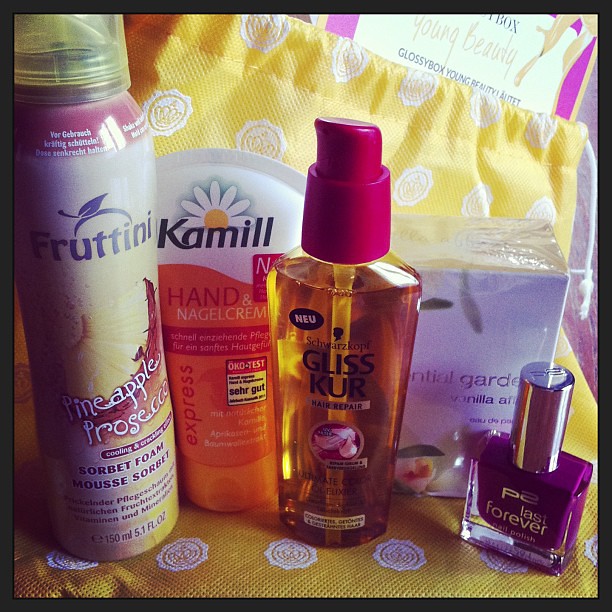In the image, a collection of beauty products and cosmetics are displayed on a tabletop, set against a backdrop that includes a yellow bag with white spots and crown designs. The image features a black frame. On the far left, there is a spray can of Frutini Sorbet Foam Mousse Prosecco, identifiable by its pineapple design and magenta lettering. Beside it, there's a tube of Camille Hand and Nagelcreme, distinguished by its orange background, daisy flower, and red lettering. Moving rightward, a clear bottle with a red spray top displays the product name Gliss Kur Hair Repair in black letters. Next to it, a white package labeled Vanilla, though mostly concealed, can be spotted. The arrangement concludes with a clear nail polish container filled with purple liquid, labeled Pierce Last Forever Nail Polish. Behind these products, the yellow bag with a cloth drawstring completes the scene.